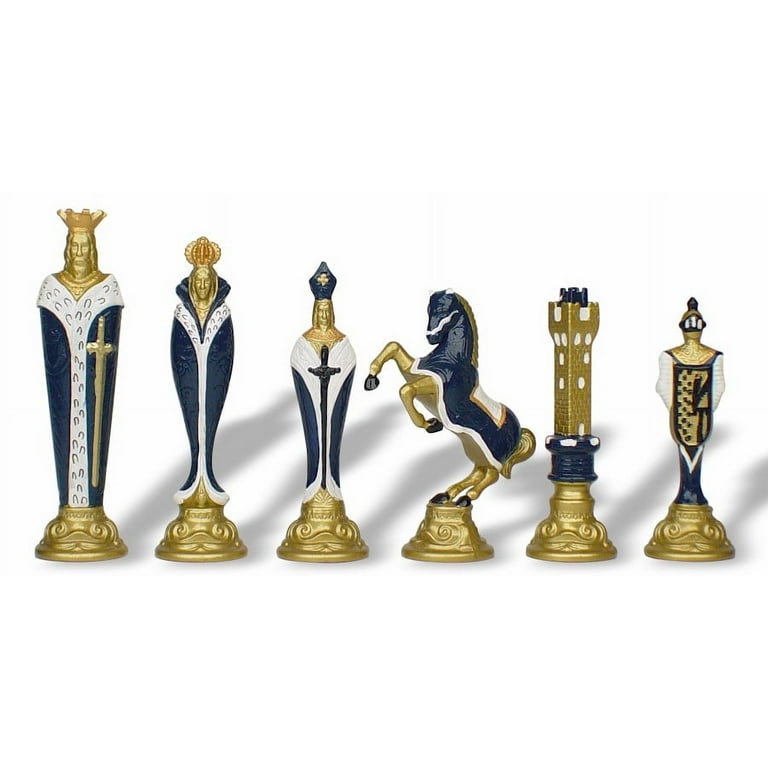The image depicts a highly detailed and seemingly rare set of chess pieces, each characterized by a sophisticated color scheme of gold, navy blue, and white. Set against a plain white background, the pieces stand in a row from left to right, casting distinct shadows to the right. The tallest piece is the king, adorned in gold, white, and blue, and depicted as an actual person. Next to the king stands the queen, also portrayed as a person and wearing a circular crown. Following the queen is a bishop, recognizable by its hat and the dagger it appears to be holding. The knight is depicted as a horse, dramatically posed with its head covered in a blue sheet and one leg kicking up high. Beside the knight, possibly representing a rook or a pawn, stands another chess piece, echoing the same elegant color scheme. The detailed craftsmanship and elaborate design make these pieces appear particularly expensive and unique.